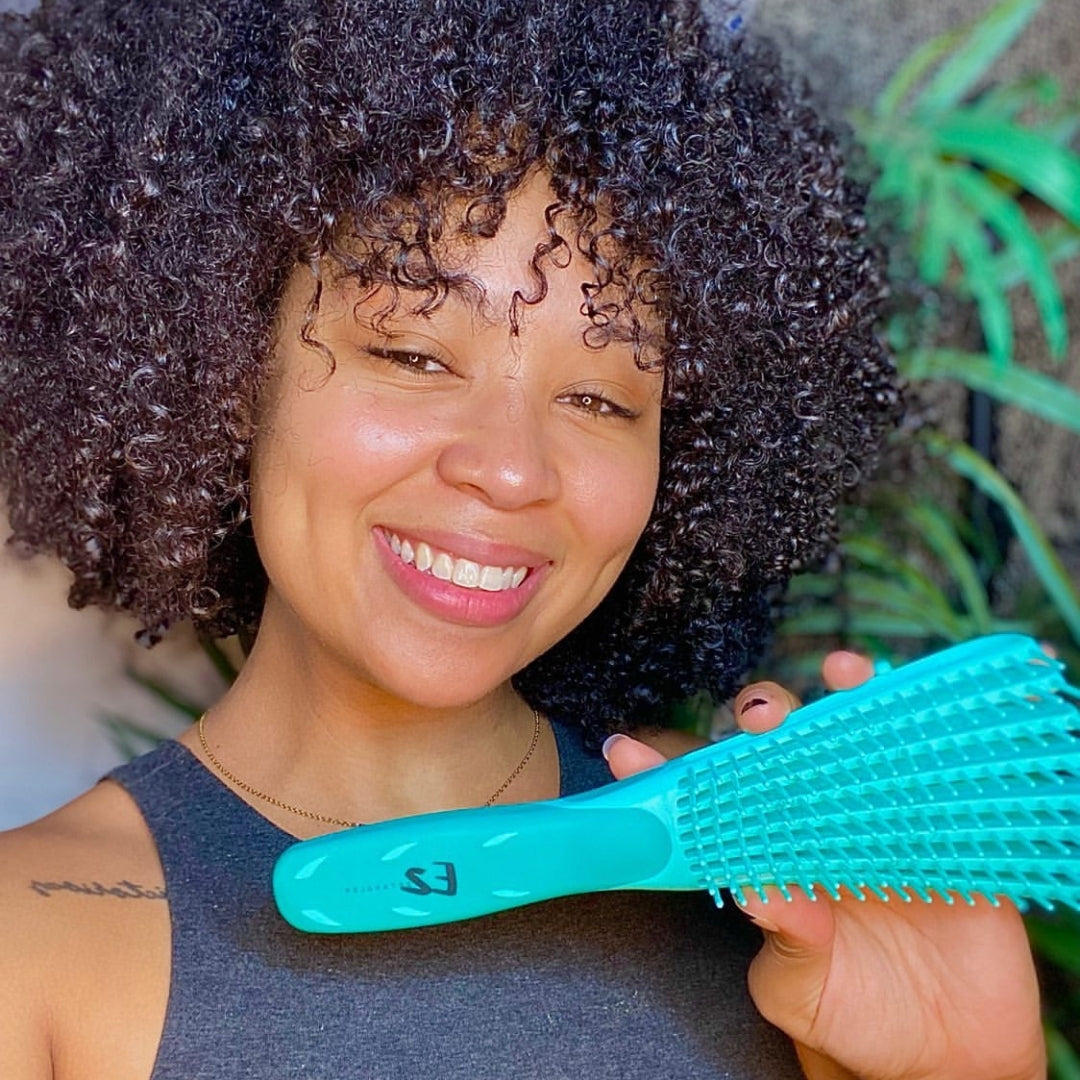The image captures a dark-complected young woman just left of center, her face and upper body taking up the majority of the frame. She has abundant, shiny, dark curly hair with tiny white highlights, cascading just above her shoulders and a few strands playfully falling on her forehead. Her head is tilted slightly to the right, showcasing a bright smile that reveals her top row of teeth. Her light brown eyes, reflecting ring lights, add a sparkle to her engaging expression, enhanced subtly by makeup.

She’s wearing a blue tank top and a fine gold chain necklace, highlighted against her darker skin. In her left hand, she holds a light blue brush by its bristled end, the handle just under her chin, while her thumb lies underneath and her other fingers curl over the top. The brush extends to the right edge of the image, partly out of frame.

A small tattoo adorns her right shoulder, barely visible due to the arm's position. The background is blurry but includes hints of green foliage, possibly from houseplants, and a darker wall to the right. Her nails are painted, contributing to the overall polished look of the portrait.